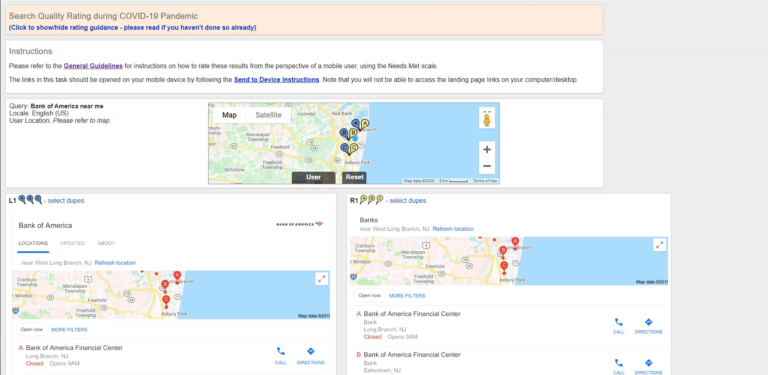The image features a gray background with a prominent pink rectangle in the center. Within this rectangle, the text "Search Quality Rating during COVID-19 Pandemic" is displayed in green. Additionally, blue text in parentheses reads, "Click to Show/Hide Rating Guidance. Please read if you haven't done so already."

Below the pink rectangle, there are detailed instructions written in purple: "Please refer to General Guidelines for instructions on how to rate. Please evaluate these results from the perspective of a mobile user using the Needs Met Scale."

The image includes a map with several location icons. The query, "Bank of America near me," is displayed in bold black text. Adjacent to this, there is locale information with "English (US)" in parentheses, indicating the user's location is within the United States, and it instructs users to refer to the map.

In the lower part of the image, there are two additional white squares. The second white square contains the text "Bank of America," with the word "locations" underlined in blue. It also includes updates about the bank's various locations, which are marked on the accompanying map with location icons specifying “Bank of America Financial Center.” To the right of the map, two blue buttons are labeled "Call" and "Direction," respectively.